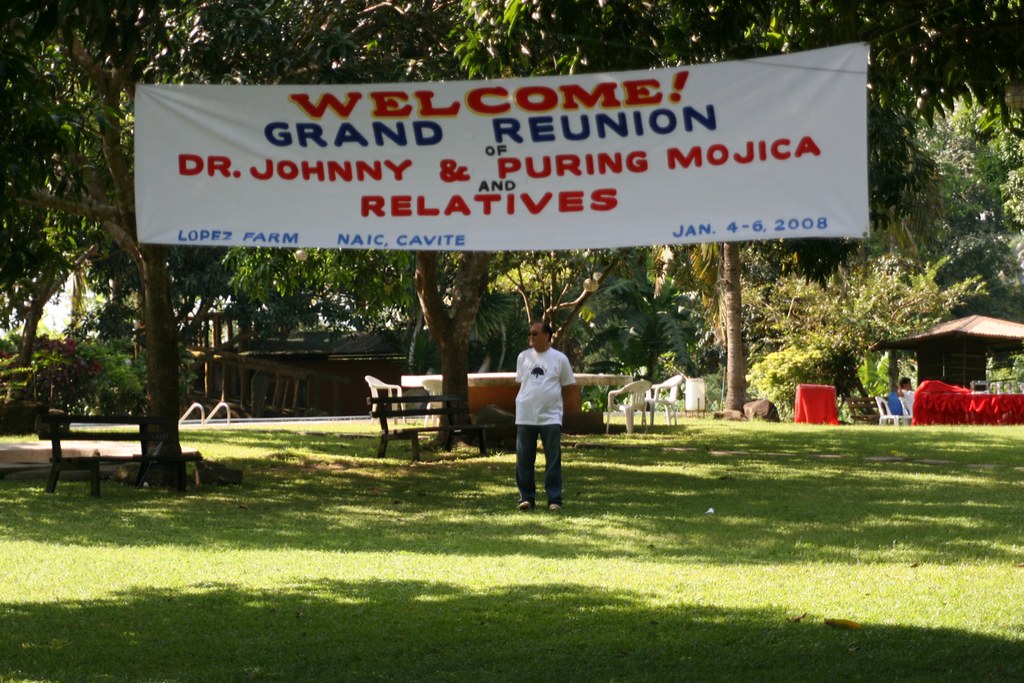This photograph captures an older man wearing a white t-shirt, dark jeans, and likely light-colored shoes, standing on a large, green grassy area in the middle of a park. The scene is bathed in sunlight, suggesting a nice, sunny day. Behind him, there's a lush backdrop filled with various trees and bushes. In the background, one can see a pool surrounded by numerous chairs and tables, some with red tablecloths and white chairs. To the right, people are seated next to a small brown building. There are buildings on both the left and right sides of the image, though they're partially obscured and difficult to identify. Dominating the scene above the man is a large white banner with red and blue text. In red font, it reads "Welcome!" followed by, in blue font, "Grand Reunion of," and then in red again, "Dr. Johnny and Puring Mojica and Relatives." At the bottom, also in blue font, it states "Lopez Farm, NAIC, Cavite, January 4-6, 2008." The man stands with his hands behind his back, offering a welcoming presence amidst the celebratory setting.